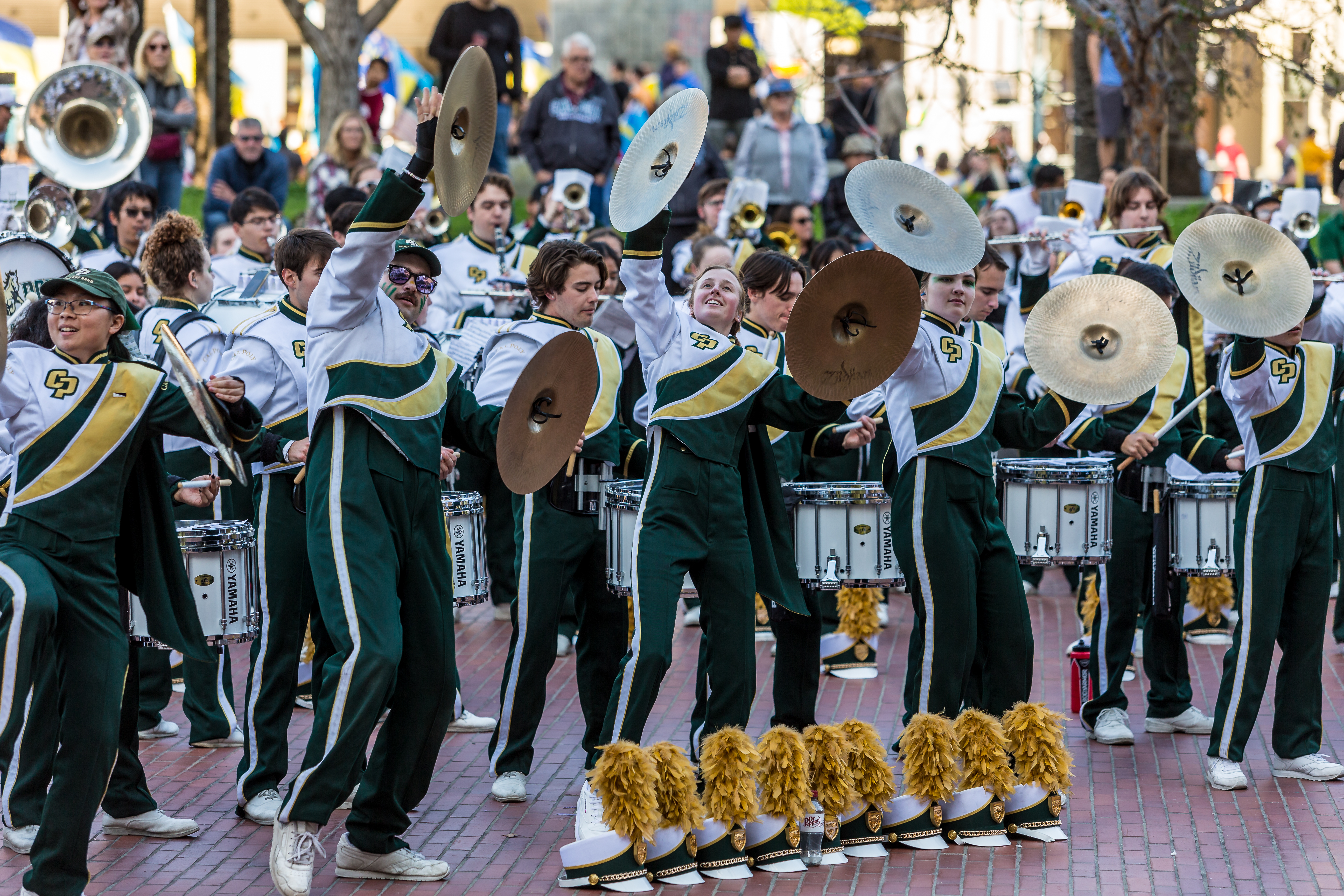The image is a vibrant color photograph taken outdoors at a public parade. In the foreground, a marching band is prominently featured, standing atop a brick-style platform. The members, clad in matching green and white uniforms, are seen performing energetically. Their uniforms consist of green pants, each adorned with a white stripe down the side, paired with white jackets accented with green and yellow details, completing their attire with white sneakers.

At the forefront of the band, the cymbal section stands out, their arms extended wide as though they have just clapped their cymbals. Four cymbal players occupy this front row, their instruments glinting in the light. Directly in front of them, neatly lined up on the ground, are their marching band hats—white with green fronts, each crowned with a distinctive mustard yellow feathered plume.

Behind the cymbal players, additional rows of band members and their various instruments create a dynamic layer, though more blurred to emphasize the depth. The background is filled with blurred figures, indicative of a lively crowd seated and standing in a park-like setting, capturing the essence of community and festivity.